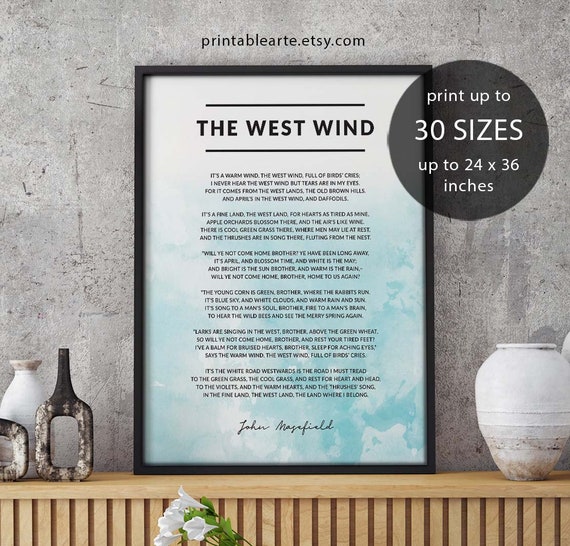This photograph showcases a beautifully arranged product display, likely intended as an advertisement for customizable prints on Etsy. Central to the image is a rectangular black photo frame that encloses a lengthy piece of prose titled "The West Wind," authored by John Masefield, as signed at the bottom. The background of the text mimics the look of clouds with a serene blend of blue and white hues.

The frame rests on a light brown wooden surface adorned with various items, including vases and pottery, adding an organic touch to the scene. The backdrop is a minimalist gray granite wall, enhancing the overall aesthetic.

Additional elements in the photo include promotional text, with "printableart.etsy.com" at the top and a semi-transparent circle on the right indicating, "Print up to 30 sizes up to 24x36 inches." This detail underscores the customizable nature of the product, emphasizing its versatility and suitability for various display needs.